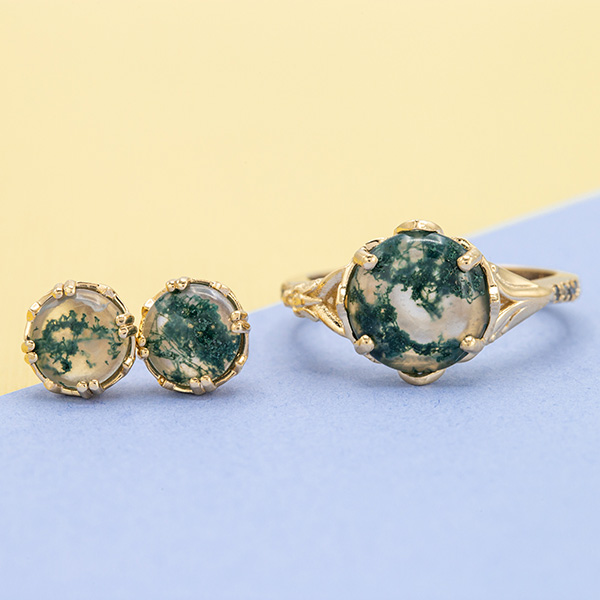The image features a set of jewelry, comprising a pair of earrings and a matching ring, showcased against a two-toned background. The lower portion of the background is a soft blue hue, transitioning into a light, soft yellow at the top. 

On the left side of the image are the circular earrings. Each earring encloses a stone that appears almost translucent, with an intricate pattern of green swirls reminiscent of dried tea leaves. These elegant stones are surrounded by a yellowish gold support frame, which features fine details resembling little arms situated at the 12, 3, 6, and 9 o'clock positions.

On the right side is the matching delicate ring, crafted from the same yellowish gold material. The ring mirrors the design of the earrings and contains a similar stone. The stone in the ring has clear and green segments, placed prominently at the top left, top right, bottom left, and bottom right corners, echoing the artistic arrangement of the earrings.